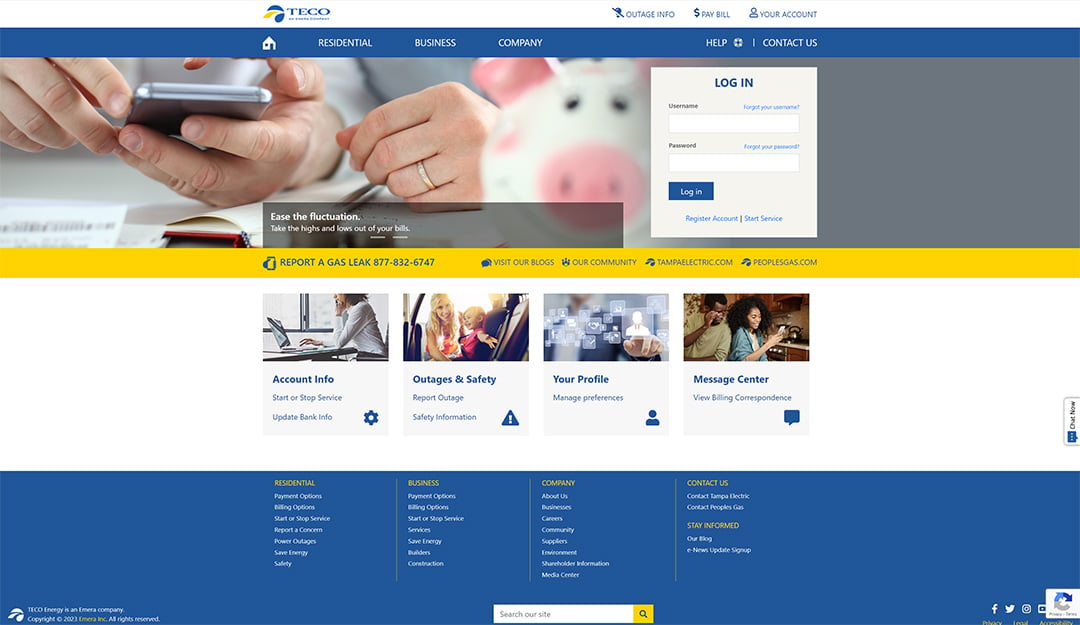This image is a screenshot of a complex web page, with numerous elements outlined in varying levels of readability:

At the very top, above the menu, the name of the company is prominently displayed in capital letters, colored blue: T-E-C-O. To the left of the company name is the company logo, which appears to be a combination of a teardrop shape at the bottom, a crescent at the top, and a small gold element resembling a flower. Beneath the logo, additional text is present but unfortunately not readable.

On the right side of the top menu, the words "Outage Info," "Pay Bill," and "Your Account" are clearly visible, suggesting the website belongs to a utility company. Below this menu, a blue header spans the page, with the words "Residential," "Business," "Company," "Help," and "Contact Us" in white font.

Beneath this header, to the left, there's a photograph depicting the hands of a man holding a smartphone. The man has light skin, likely indicating he is either white, Asian, or Hispanic. Next to the man’s hands is the left hand of a woman with similarly pale skin, wearing a gold ring that is probably a wedding ring. The image is slightly out of focus, but a white ceramic piggy bank with a prominent pink nose is also visible.

To the right of the photograph, there is a login screen within a gray square. At the top of this section, the word "Login" is displayed, followed by two white rectangles meant for entering a username and password. Beneath these fields, a small blue rectangle presumably serves as the login button.

Further down the page, a yellow line divides the sections, beneath which another menu is presented in blue text. It includes options such as "Report a Gas Leak" with an accompanying phone number, "Visit Our Blogs," "Our Community," and two other items that are not entirely readable.

In the central portion of the page, the background is white and showcases four color photographs of individuals. 

At the very bottom of the page, the footer features a blue background with four columns of white text. The font in these columns is very small, making the text difficult to decipher.